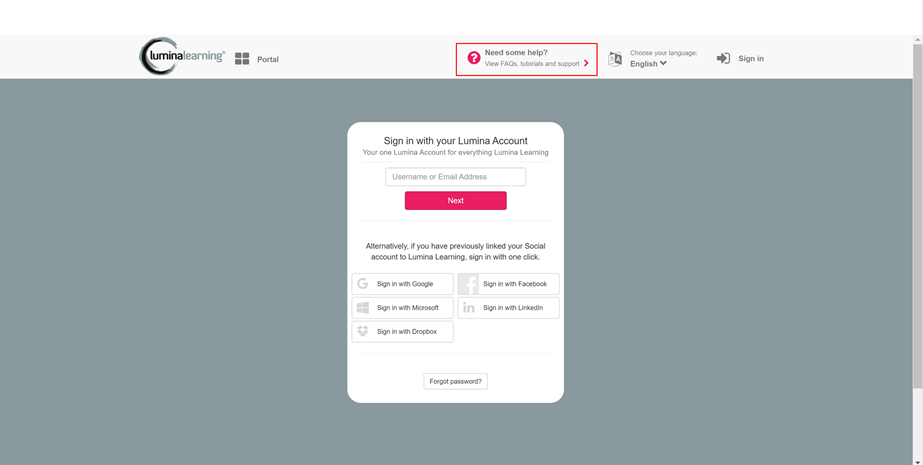The image is a screenshot of the Lumina Learning portal interface. Central to the screen are four distinct sections: "Need some help? View FAQs, tutorials, and support." These sections are highlighted with a red rectangle. Adjacent to this, there is a pink circle featuring a white question mark. The top-right corner of the screen displays a language selection option, with English currently selected. Near this, there are two options: "Sign in" and a square icon with an arrow pointing into it, indicating the sign-in area. There is also an option to sign up with your Lumina account, which reads, "One Lumina account for everything Lumina Learning." Below this, a text box is available for inputting a username or email address. A rectangular button, shaded in a reddish-pink color and labeled "Next" in white letters, is situated beneath the text box. An additional note indicates that if the user has previously linked their social account to Lumina Learning, they can sign in with a single click.